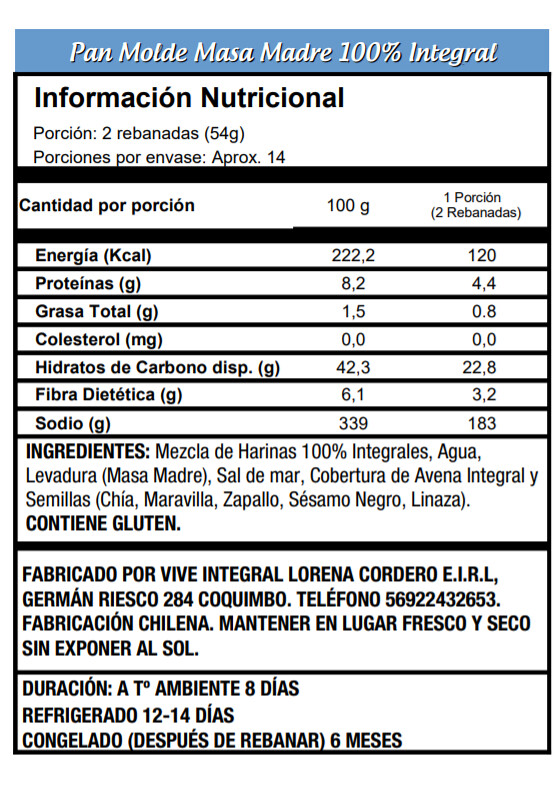This image features a detailed nutritional label in Spanish, predominantly in black and white. The top portion of the label boasts a striking blue background with white text that reads "Pan Molde Masa Madre 100% Integral." Below this, the label follows the conventional format of nutritional information, beginning with "Información Nutricional" and specifying that the portion size is "2 Rebanadas" (54 grams), with approximately 14 portions per package.

The label provides comprehensive statistics similar to those found on English labels, listing details such as Calories ("Energía"), Protein, Cholesterol, Carbohydrates, Fiber, and Sodium. Also included are instructions for refrigeration and storage duration. The ingredients list highlights that the product is made from "mezcla de harinas 100% integrales" (a mix of 100% whole grain flours), along with other components like "agua, levadura masa madre, sal de mar, and a variety of seeds such as chia, sunflower, pumpkin, sesame, and flax seeds." It is noted that the product contains gluten.